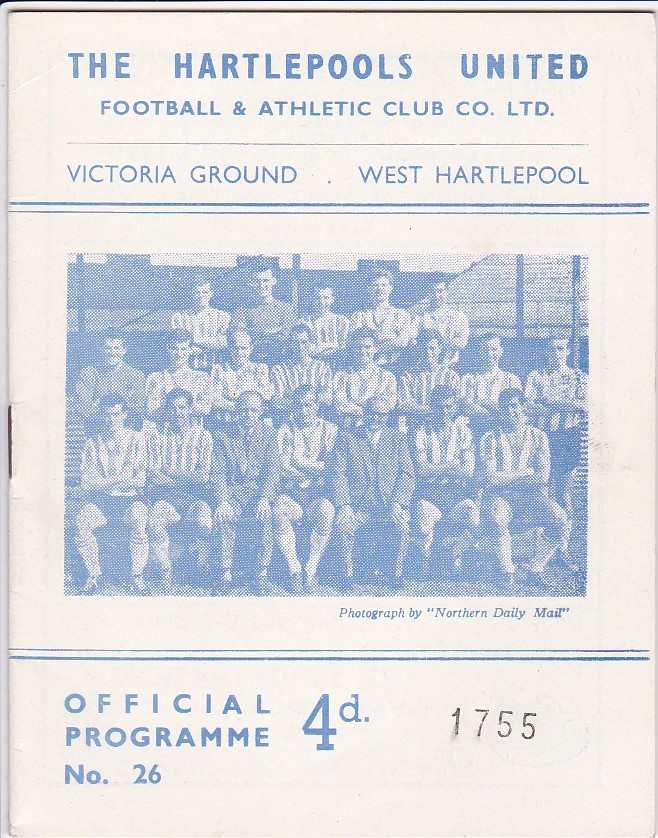The image is a vintage match program printed on light white paper, likely cardstock, featuring blue text and images. At the top, it prominently displays "THE HARTLEPOOLS UNITED" in blue capital letters. Below this, in slightly smaller letters, it reads "Football and Athletic Club Company Limited." A horizontal line separates this from the text "VICTORIA GROUND" followed by "WEST HARTLEPOOL," all in capital letters. Beneath are two horizontal lines, one dark blue and one lighter blue. 

The center of the cover is occupied by a picture of the football team, although it's somewhat unclear and lined. The team photo consists of three rows of men; the coach and manager, identified by their suits, sit in the front row, while the rest of the team is dressed in kits. Below the photo, in small font, it says "Photographed by 'Northern Daily Mail'." Two more lines, one lighter and one darker, run underneath this caption.

In the lower segment of the cover, the word "OFFICIAL" is printed on the left side, followed by "PROGRAM," and then "NUMBER 26." To the right, an indication of price as "4D." On the bottom right-hand side, it is stamped "1755," possibly denoting the edition number or the number of copies printed.